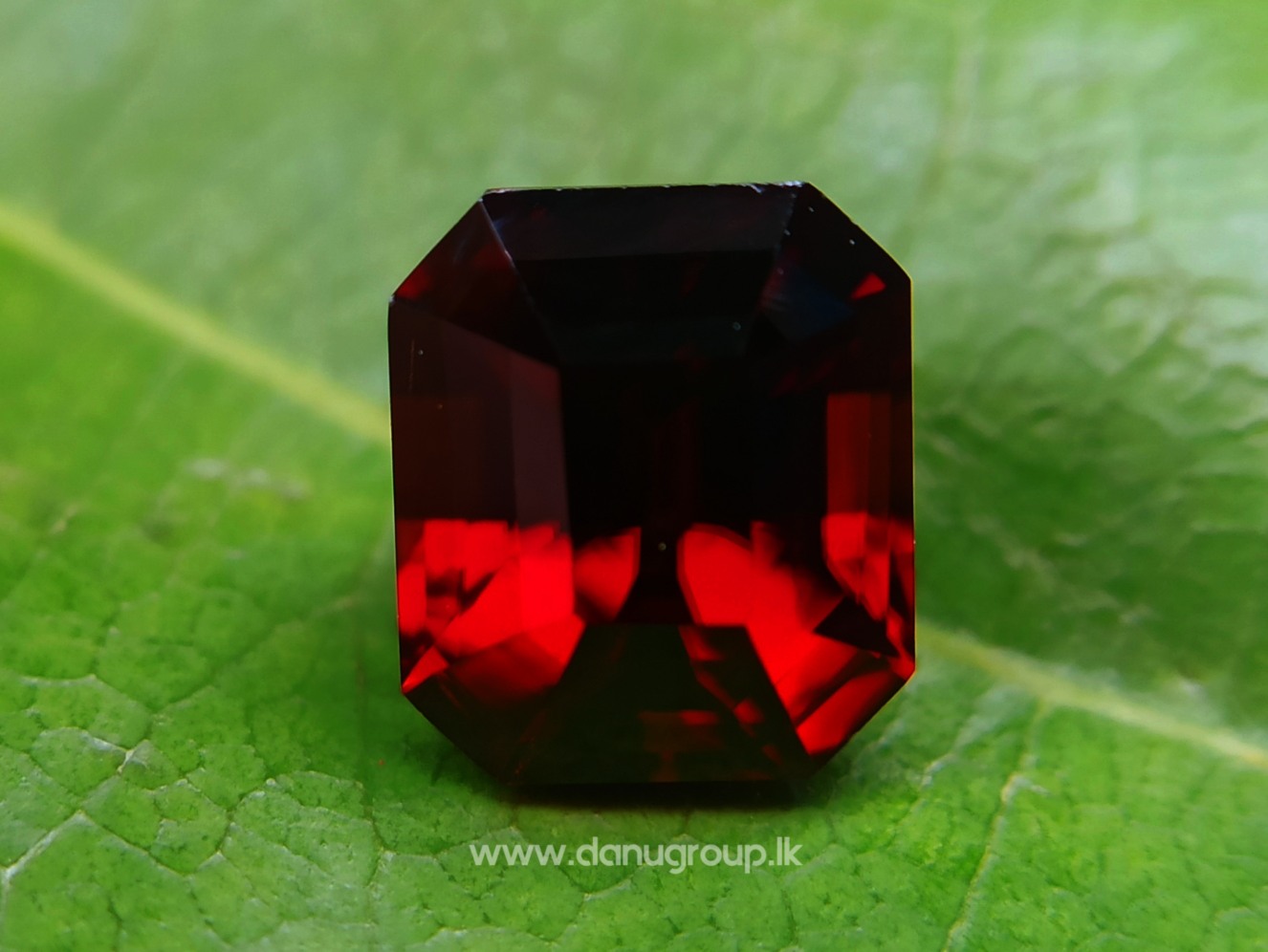A close-up image captures a rectangular-cut gemstone, likely a ruby or garnet, with beveled edges. The gem transitions from almost black at the top to a glowing red in the middle and darkens again towards the bottom, influenced by the light. The stone rests on a vibrant green leaf with yellowish hues and distinct veins. The background fades out at the top, putting full focus on the gem. At the bottom, white text reads "www.danugroup.ok."